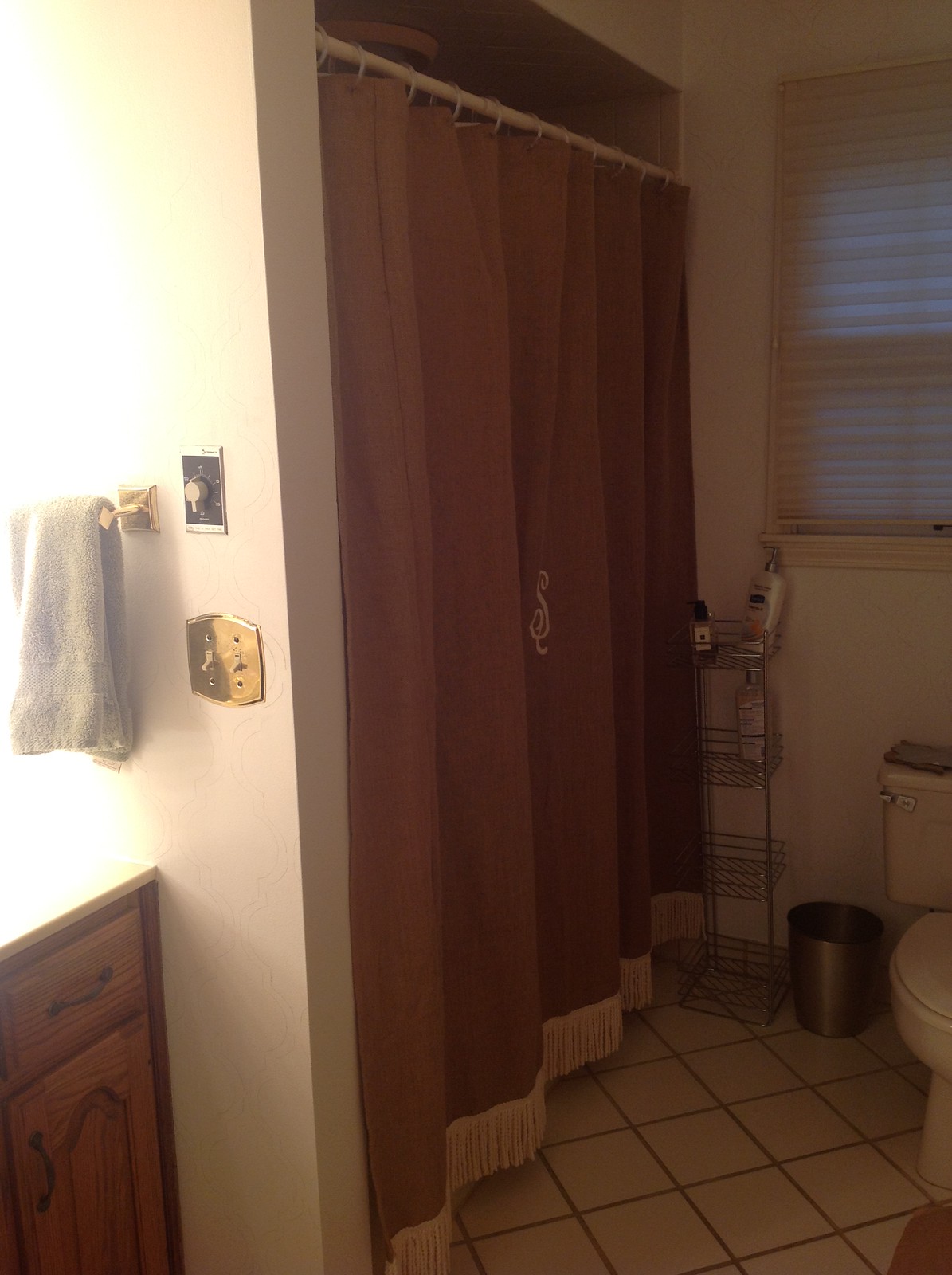This is a detailed portrait mode photograph of an interior bathroom. Dominating the center of the image is a dusty brown shower curtain with a cursive embroidered 'S' near the top, and a white fringe border at the bottom, hanging on a white rod with clear or white rings. On the left-hand side, a dim light shines brightly from the vanity light, slightly washing out a towel rack that holds a light gray or light blue towel. Below the towel rack, a black background timer with a cream-colored dial is mounted on the wall, alongside a brass light switch plate with two small white switches. The walls are painted white.

Further left, an old wood vanity cabinet, dating back to the 1970s or 1980s, has visible wood drawers and doors all with handles, and a white countertop, though most of it is cut off from view. Towards the right-hand side, partially in view, is a white toilet with a silver handle, adjacent to a shiny metal trash can. Alongside the toilet stands a multi-tiered metal rack holding bottles of lotion and other toiletries. The back wall features a small window with white blinds, allowing a glimpse of blue sky from outside. The floor is tiled in a cream and brown checkered pattern with contrasting brown grout, and a small pink rug is laid out over the tiles.